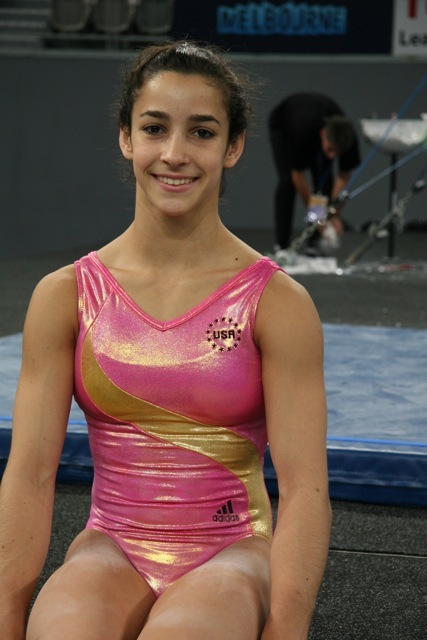The image depicts a young female gymnast with tan skin and short brown hair styled in an updo. She is seated on a gray carpeted floor, with her knees partly visible at the bottom left of the photograph. She's smiling widely, showing her top teeth, and exudes a friendly, confident demeanor with her dark brown eyebrows complementing her expression. 

The gymnast is wearing a striking bright pink sparkly leotard adorned with a gold swirly pattern. The leotard features a V-neck with thick shoulder straps and prominently displays two logos: a black "USA" with surrounding stars on the chest and an Adidas logo higher up on the thigh area. Her thighs are notably dusted with chalk, hinting at her readiness for competition.

In the background, the floor is visibly set for gymnastics, marked by a blue padding used for floor routines. A man dressed in black shirt and pants is absorbed in attending to some wires, perhaps adjusting some gymnastics equipment. The setting appears to be indoors, with a sign saying "Melbourne" visible further enhancing the competitive ambiance.